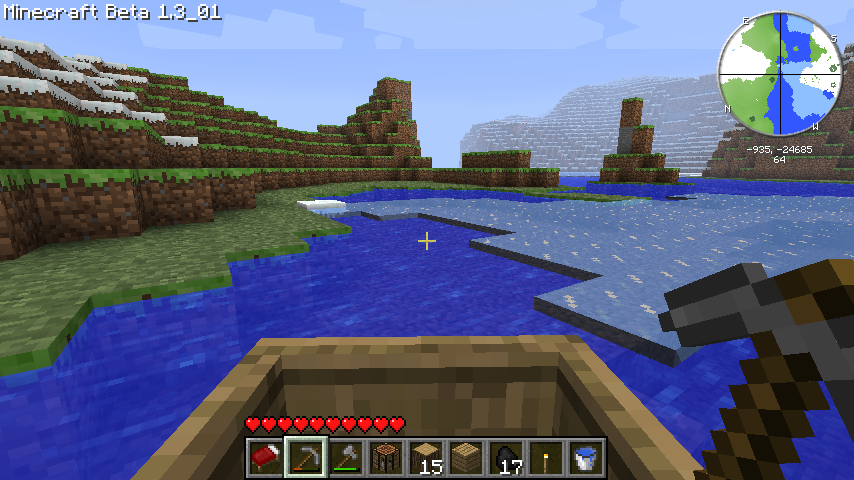This is a detailed screenshot of the video game Minecraft in its Beta 1.3_01 version, as indicated at the top left corner of the screen. The game is displayed in its iconic blocky, pixelated style, with each element rendered as cube-like structures. The first-person view shows the player's perspective, including their pixelated pickaxe tool held out. The scene appears to place the player inside a small, brown boat floating on a blue, cubed lake surrounded by green terrain. In the distance, there are rocky and snowy mountains, also constructed from cubes, and even the clouds in the blue sky are square-shaped.

On the top right corner of the screen, there is a circular compass displaying the directions North, East, South, and West, with coordinates beneath it reading -935, -24685, and a value of 64 which might denote elevation. At the center of the screen, a small cursor is visible, suggesting the player's focus point. At the bottom of the screen is a toolbar showing at least ten different tools or items available for the player to use. Above this toolbar, ten heart icons display the player's health status. The image captures the quintessentially blocky, creative, and exploratory essence of Minecraft.